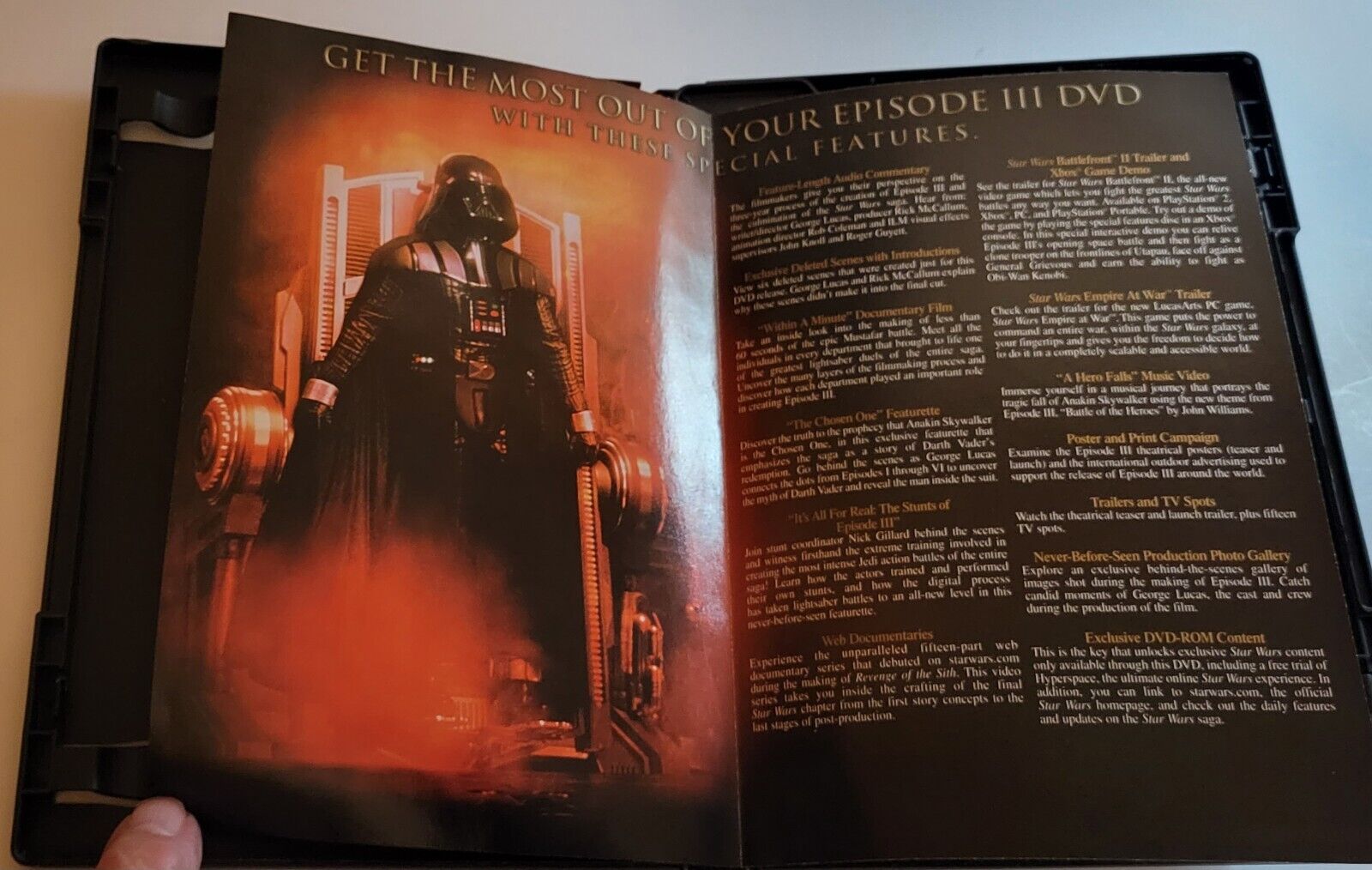The photograph captures a close-up of an open DVD case for "Star Wars: Episode III." Within the case, there's a detailed paper insert securely held by black clips. The left side of the insert prominently features a striking image of Darth Vader in his signature black armor, complete with a full-helm, chest armor, and a control panel adorned with red buttons. He stands authoritatively on a platform or in front of a throne, surrounded by red and orange mist. Above Darth Vader, in bold gold text, it reads, "Get the most out of your Episode 3 DVD with these special features." The right side of the insert contains several paragraphs arranged in two columns, each with titles in gold text, highlighting various features of the DVD including trailers, a music video, and campaign details. The overall setup of the case’s interior, including the clips and the clasp mechanism, is also visible. Additionally, the finger of the person holding the case is seen in the bottom left corner, offering a sense of scale and interaction with the object.